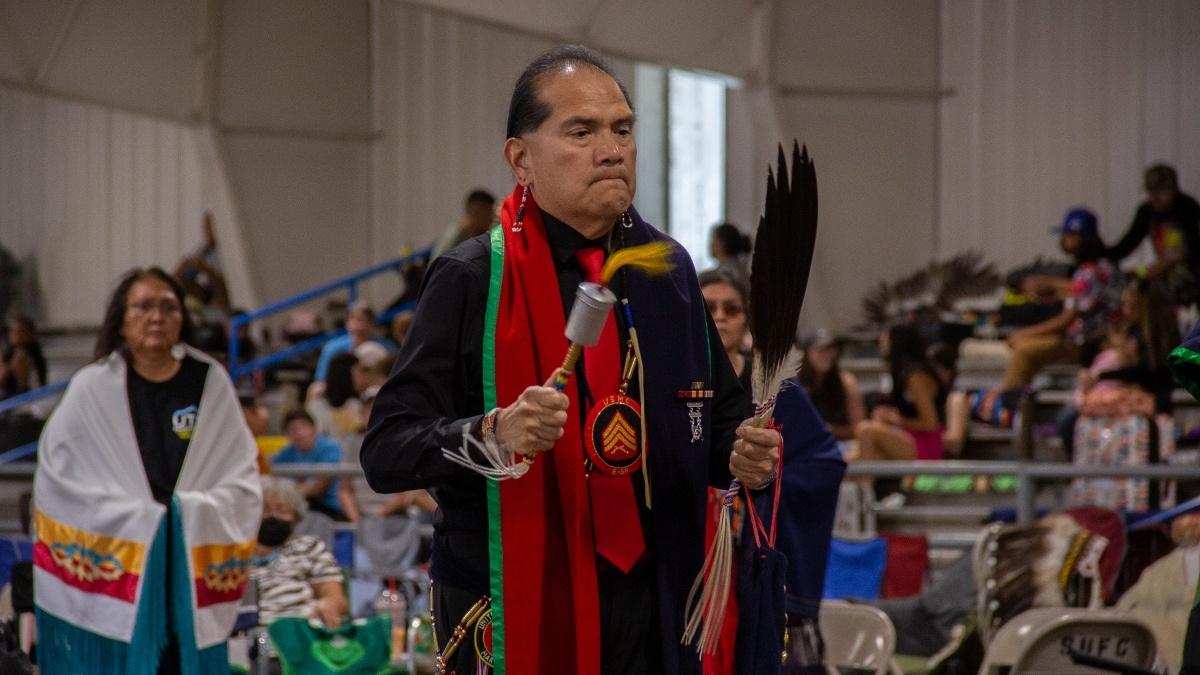This photograph, taken indoors at a ceremonial event, features a central figure believed to be a Native American man. He has light brown skin and short black hair pulled back with a receding hairline. He wears beaded earrings that dangle past his chin and is dressed in a long-sleeved black top and pants. Draped around his neck is a sash: on his right side, it’s red with a green ribbon on the outside; on his left, it's dark blue with a green ribbon. He also wears a red tie adorned with a round emblem bearing the United States Marine Corps insignia and his military rank insignia featuring three gold chevrons and crisscrossed guns.

In his left hand, the man holds a black feather with a white tip near the base. In his right hand, he grips a rattle with a handle and a gray cylindrical end decorated with red and yellow feathers. His expression is concentrated, lips pressed together.

Behind the man and slightly to his left, a woman of Native American descent stands. She has shoulder-length dark hair, wears glasses, and is dressed in a black shirt with a white frock that features blue fringe and red and yellow emblems near the bottom. Further to the left and right in the background are seated and standing spectators, some on metal bleachers. The venue is a gray metal building, with a door on the left side that lets in sunlight. Visible just past the woman are additional people, including another elderly woman with gray hair and glasses, barely discernible as she is partially obscured.

In the photo's foreground, specifically in the bottom-right corner, there’s a gray railing extending to the left and the back of a chair with black writing. The ceremonial setting and the people involved suggest a significant cultural and possibly military honoring event.